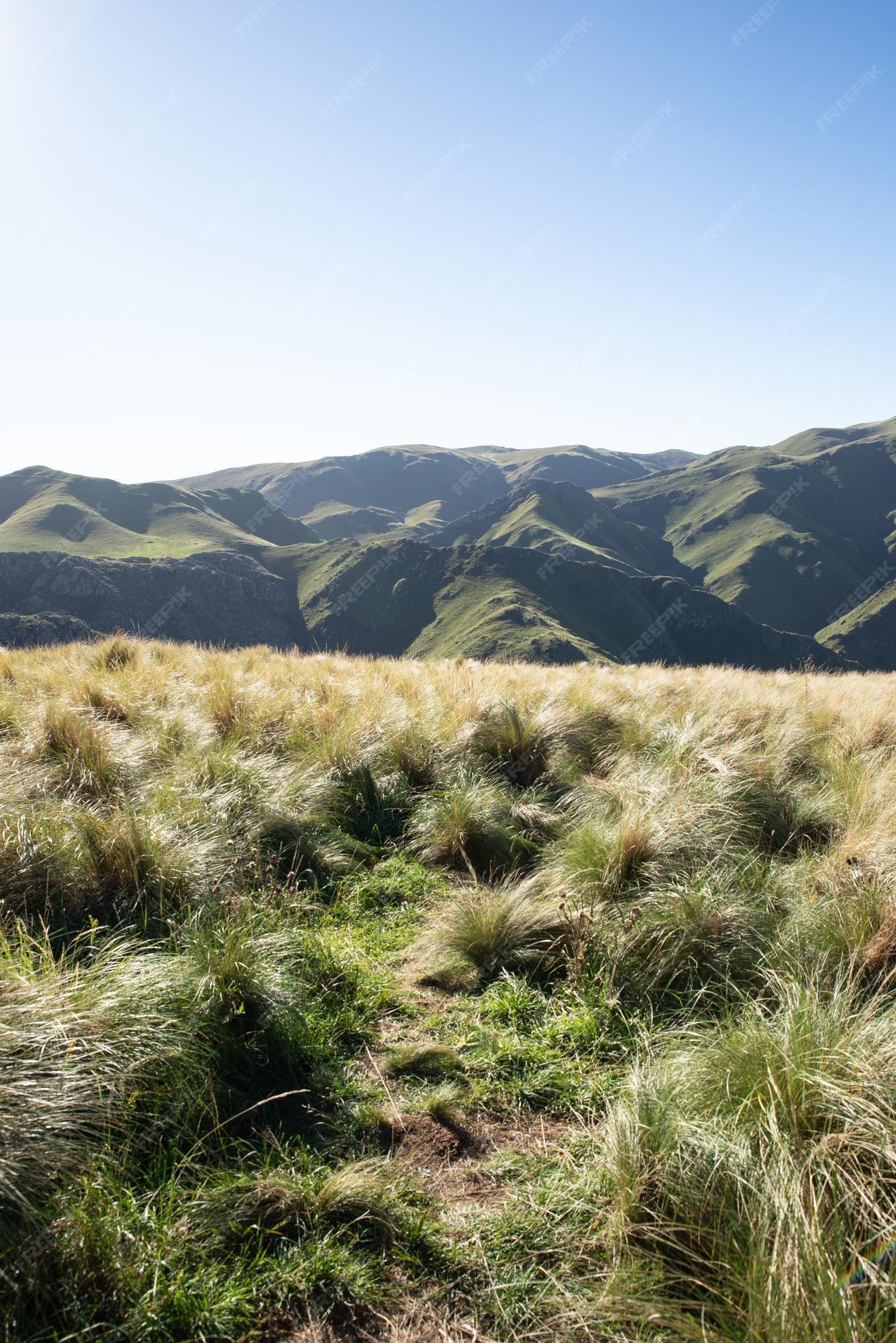This photograph captures a stunning daytime view of a mountainous landscape. Above the rugged, bumpy mountain range, the sky transitions from a dark blue in the top right to a bright, almost white hue as you move down and left. The foreground is a mixture of grassy plains with tufts of green and gold grass, along with patches of visible dirt. The scene is bathed in clear, sunny light. Notably, the image includes watermarks, possibly indicating "free pics" or similar, which slightly obfuscate some details. A faint fog can be observed in the distance, adding a touch of mystique to the serene and organic scene.